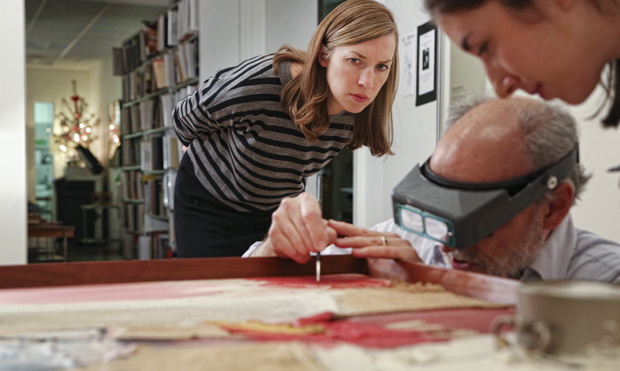In this detailed indoor color photograph, an older man is crouched over a wooden table, intensely focused on a project. He wears magnifying goggles and holds a thin, pen-like instrument, possibly a paintbrush or stylus, in his right hand. The man is balding, with gray hair on the sides of his head and a matching gray beard. His attire includes a button-up collar shirt. To his left, a woman with long blonde hair and dressed in a black and gray striped shirt leans over, closely observing his work. She appears slightly blurred in the background. On his right, another woman stands in clear focus, watching attentively. The background showcases a bookshelf filled with numerous books, white walls, and additional hints of an adjacent room, which includes a small bear Christmas tree on a table in the corner and a gray coffee mug on a lower surface. The ambient setting is bright, highlighting the concentration and collaboration in the scene.